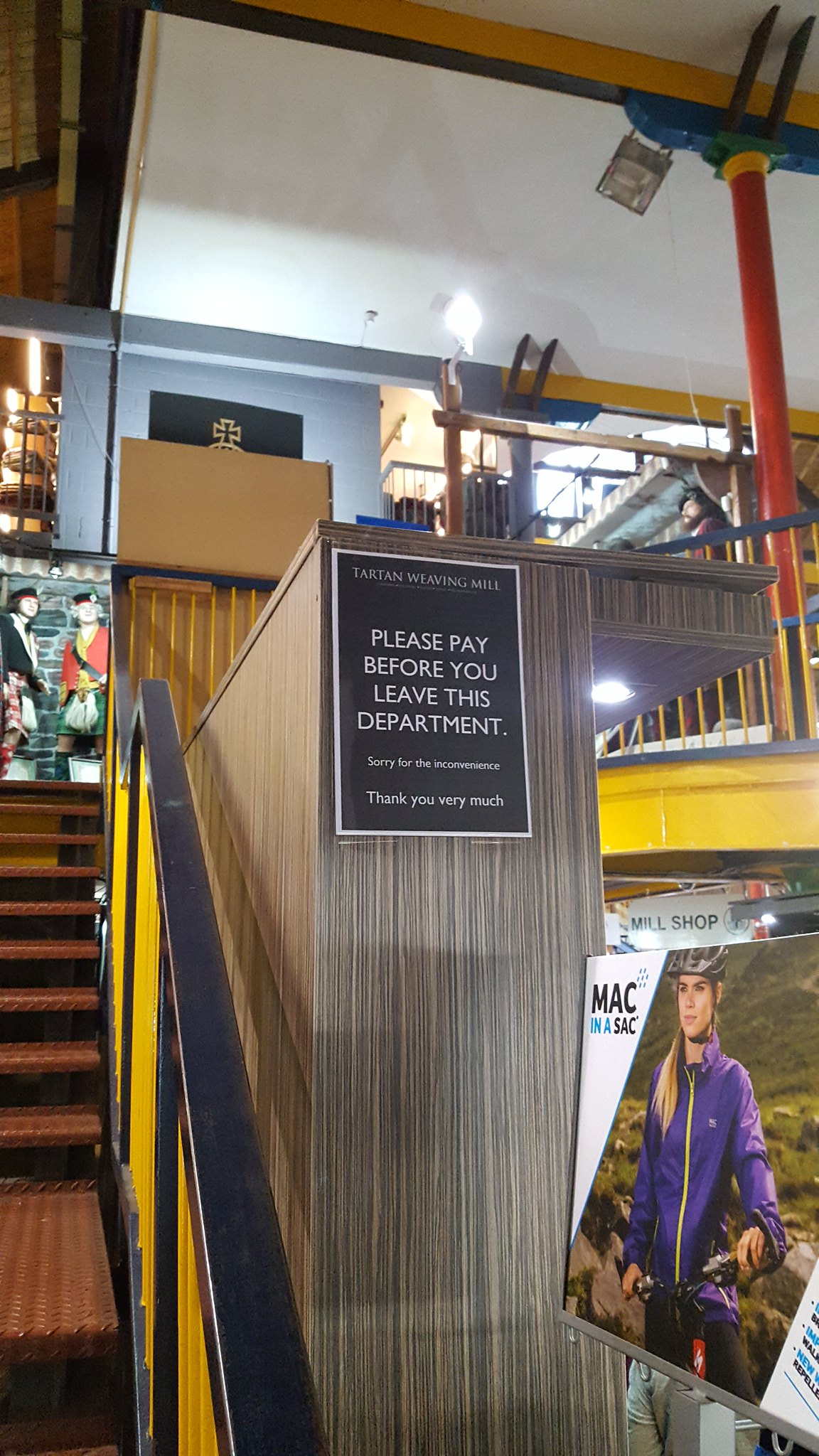The image captures the interior of a store named Tiffany Mall. Dominating the center is a black poster with white text, reading, "Please pay before you leave this department. Sorry for the inconvenience. Thank you very much." The lower section of the poster also mentions "Charton Weaving Mill." The scene features a staircase with a black handrail and yellow accents, leading to the upper floor which has white walls on top and blue walls on the bottom. Along the stairway, there's a picture of two people dressed in traditional costumes, and a black poster hangs nearby. On the lower right side of the image, there's a poster of a woman on a bicycle, wearing a helmet and a purple jacket, labeled "Mac in a sack." The environment includes wooden walls, a red pole with a light, and another light illuminating the wall. Additionally, mannequins in traditional attire are displayed on the upper floor. The overall composition has a somewhat cluttered and eclectic feel, with various elements drawing the eye.